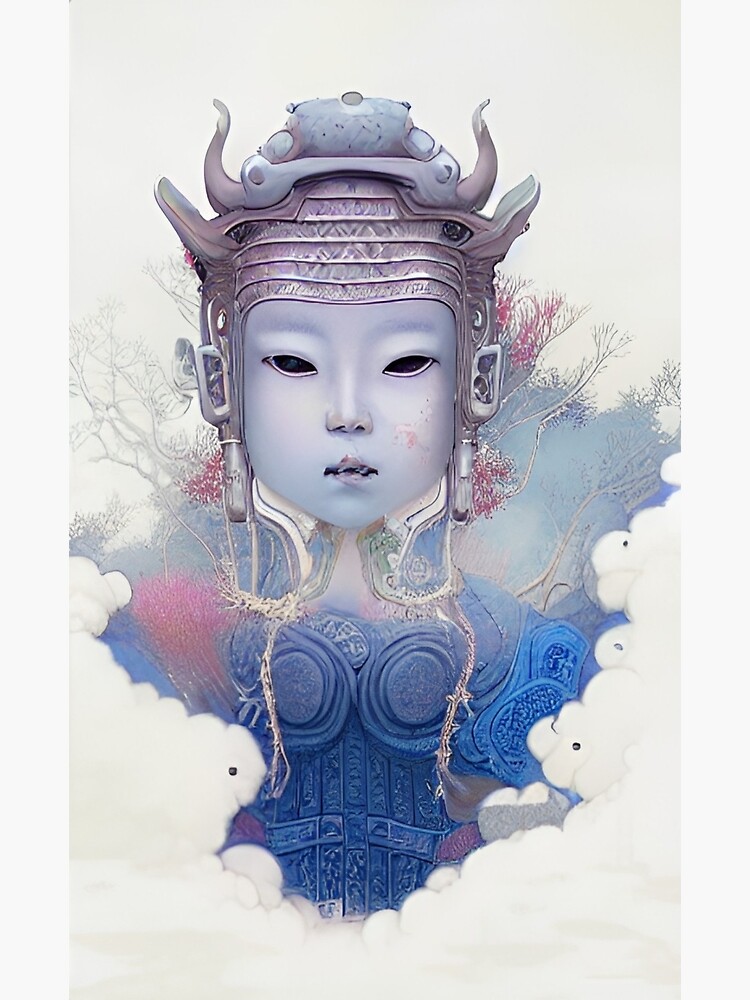This image is a detailed, computer-generated digital illustration depicting an otherworldly, almost deity-like figure with an intricate and haunting appearance. The central figure is an Asian woman with completely black pupils and extremely pale, almost gray skin. Her lips are an unusual, broken-up gray rather than a natural color, contributing to her eerie look.

She dons an ornate, elaborate headdress that appears to be made of metal, with a blend of brown and violet hues matching her skin tone. The headdress is adorned with four prominent horns—two curving to the sides and two extending upwards—enhancing her otherworldly presence.

Her attire resembles ancient armor or a military-style uniform, mainly in a striking blue color. It includes high collars and round padded sections on her chest, suggesting protective gear. This blue armor appears to be intricately ornamented and almost melds into her form.

Surrounding her, the background is filled with fantastical elements: white trees with red leaves grow behind her, surrounded by clouds and vines that drape over her shoulders. The lower half of her body is obscured by swirling clouds of smoke or steam, adding to the mystical and surreal atmosphere of the scene. All these details combined create a vivid and bizarre image of a spirit or mythical figure enveloped in a spectral, enchanted forest.